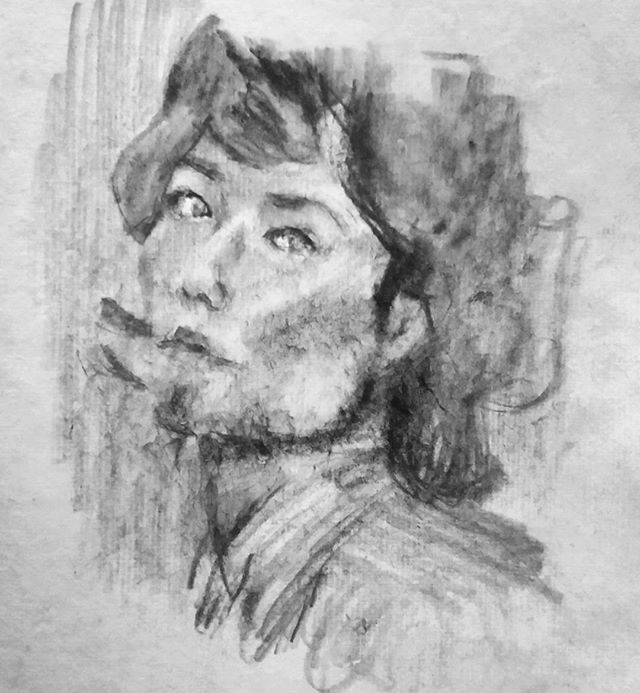This next image showcases a meticulously detailed pencil drawing in black and white, depicting the face of a woman. She gazes sideways toward the viewer, seemingly engaged with the artist. Her hair cascades down and touches the top of her shoulders, with strands falling naturally onto her forehead. Her neck is visible, emphasizing her high cheekbones and well-defined eyebrows. The artist has taken a free-form approach with the drawing, ensuring her facial features are clear and precise, while her hair is rendered in a more abstract manner with expressive strikes of the pencil. This contrast adds a dynamic and spontaneous quality to the artwork.